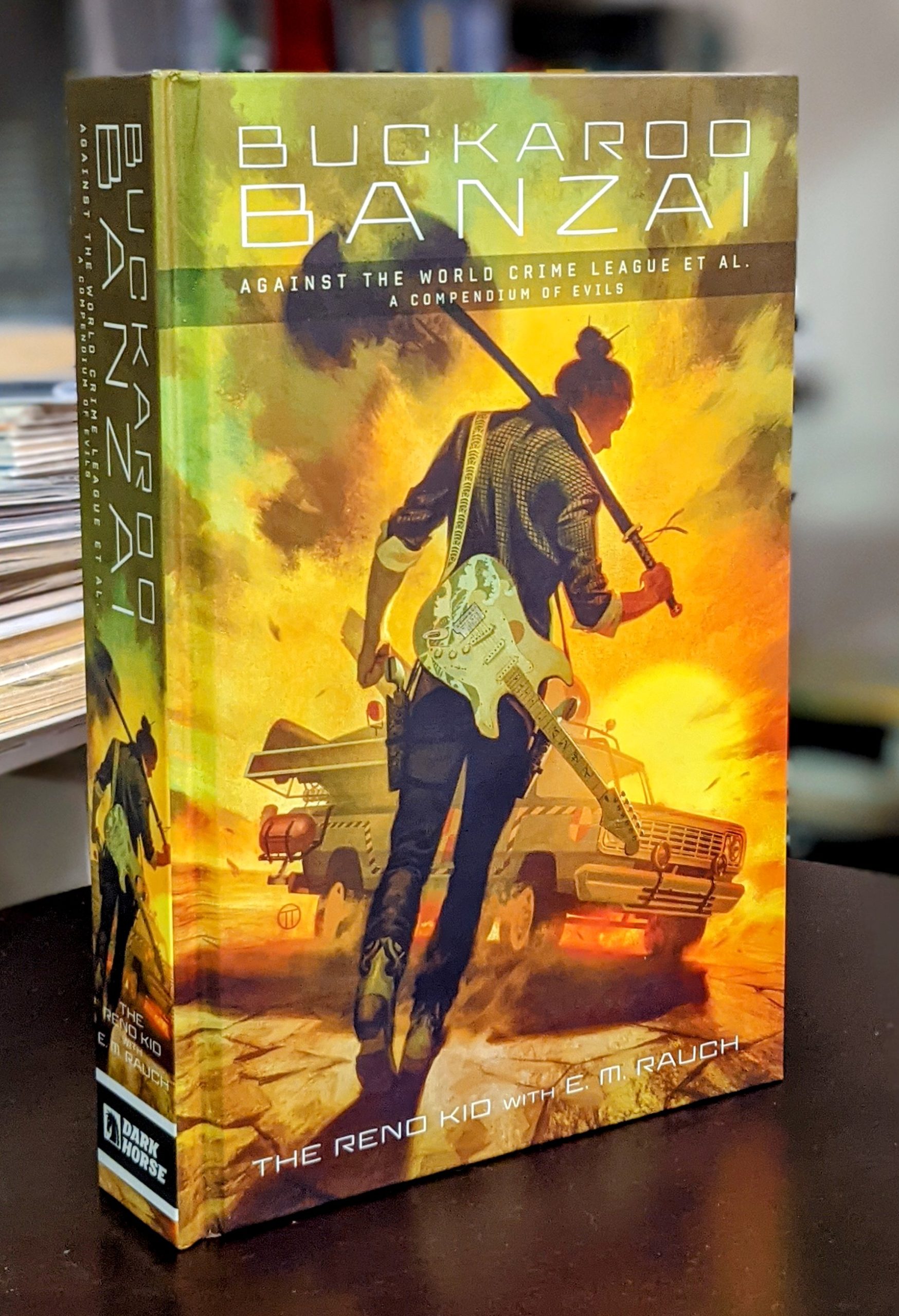This professionally staged, vertically rectangular, full-color photograph showcases the front cover of a hardback book titled "Buckaroo Banzai Against the World Crime League et al., A Consortium of Evil." Photographed indoors with artificial lighting, the image is free of any specific background and stands upright on a shiny, polished dark brown table that reflects the book's image.

Dominating the cover is a striking illustration featuring a man with his back slightly turned to the viewer, accentuated by a fiery sunset filled with swirling clouds. He is outfitted in dark pants and a black and white checkered shirt with rolled-up sleeves. Over his right shoulder, he carries a sheathed samurai sword, while a guitar is slung across his back, the neck pointing downwards. His hair is tied up in a bun, and he has a holstered gun on his left hip.

To the right of the man, a military-style jeep or possibly a semi-truck vehicle is seen driving under the backdrop of a brilliant yellow and orange sunset. At the book's bottom, the text reads "The Reno Kid with E.M. Rauch," denoting the author. The spine of the book, partially visible, mirrors the cover’s orange-yellow hues and includes the same title and a smaller version of the man’s figure, along with the publisher's mark, "Dark Horse."